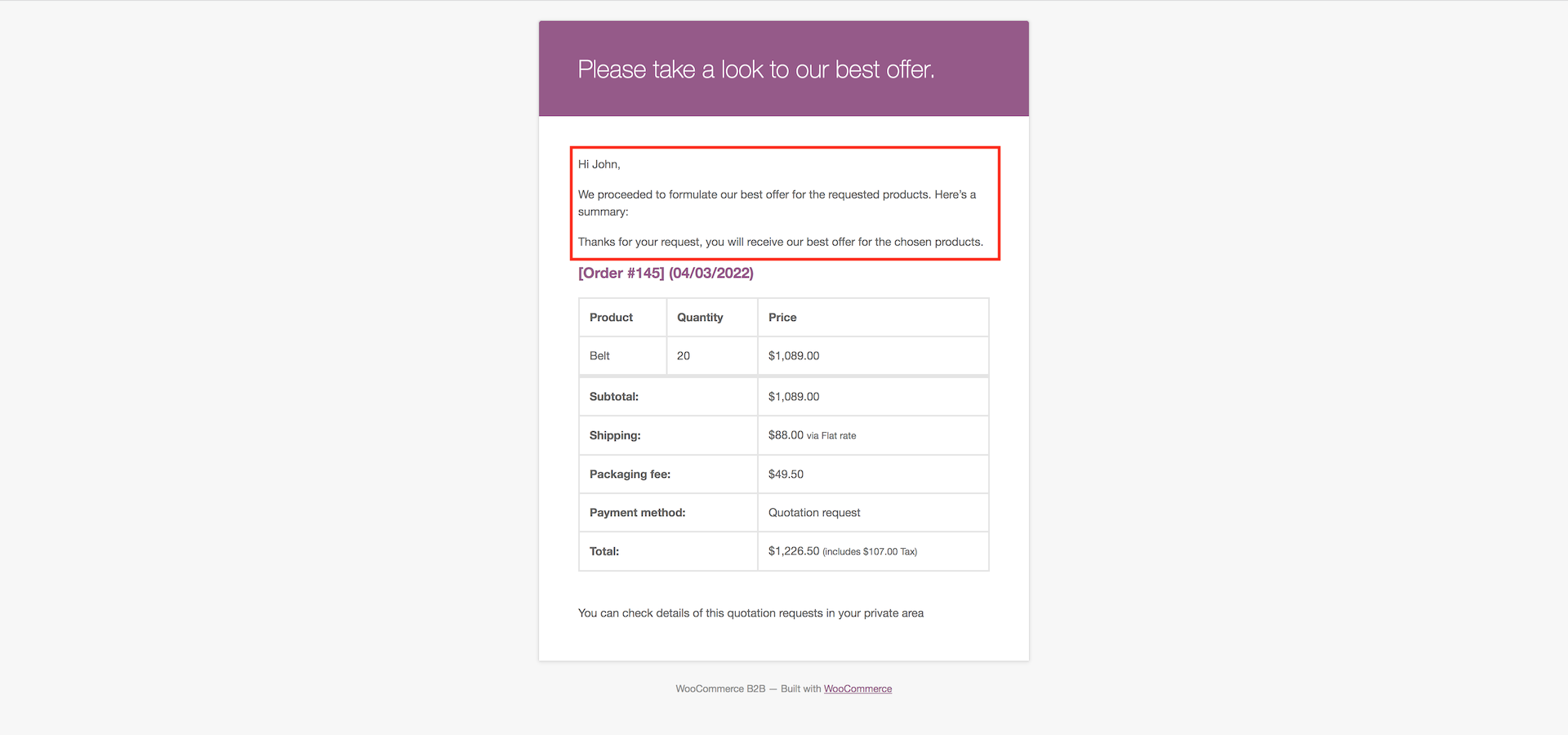The screenshot features a light gray background with a central white rectangle that is slightly taller than it is wide. At the top of this rectangle is a purple-bordered header, containing the text "PLEASE TAKE A LOOK AT OUR BEST OFFER" in white letters.

Below the header, within a red-outlined white section, the text reads: "Hi John, we proceeded to formulate our best offer for the requested products. Here's a summary. Thanks for your request, you will receive our best offer for the chosen products."

Following this message is a line of text, in purple: "Order Number: 145 (04-03-2022)." Beneath this, there are three columns labeled "Product," "Quantity," and "Price."

The breakdown of the order is as follows:
- Product: Belt
- Quantity: 20
- Price: $1,089

The section concludes with a summary of costs:
- Subtotal: $1,089
- Shipping: $88
- Packing Fee: $49.50
- Payment Method: Quotation Request
- Total: $1,226.50